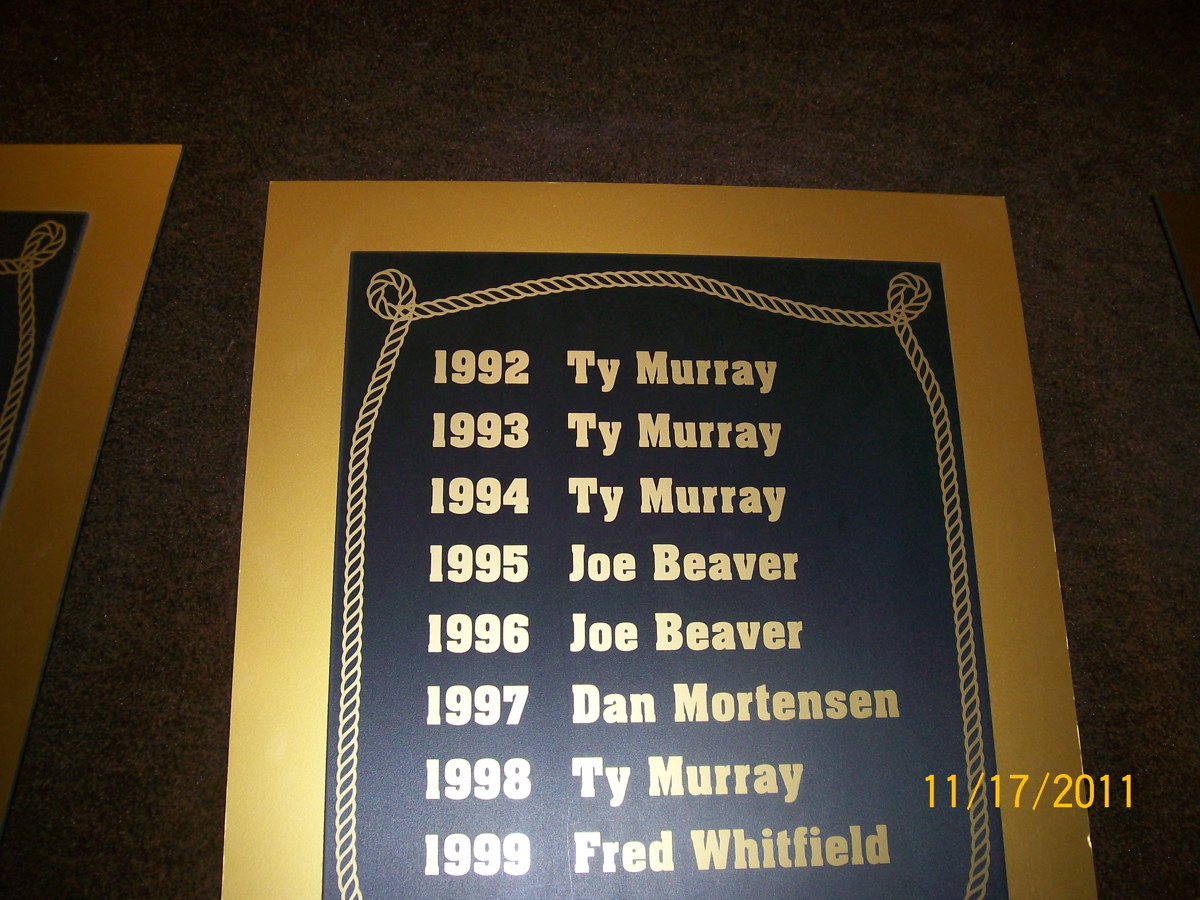The image features a centrally positioned sign against a dark fabric backdrop, possibly a wall or floor, creating an indoor, dimly lit ambiance reminiscent of a sports museum. The sign is bordered with a wide gold frame and has an inner design resembling a thick rope. The main body of the sign is black with gold text listing notable names and years: Ty Murray is listed multiple times (1992, 1993, 1994, 1998), Joe Beaver appears twice (1995, 1996), Dan Mortensen is mentioned for 1997, and Fred Whitfield for 1999. The bottom right corner of the image shows the date "11/17/2011" in yellow text. The scene captures a nostalgic and commemorative atmosphere with dominant hues of brown, yellow, dark blue, and gold.